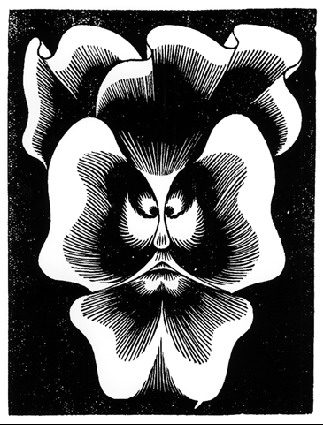The image is a tall, rectangular black and white artwork, possibly a print or pen drawing, with a thin white border. The background is completely black with several tiny white and gray specks scattered mainly around the corners and edges. At the center of the composition is a detailed drawing that appears both floral and human. The central image closely resembles a pansy or a set of curved and folded petals, drawing the viewer's eye to the intricate face formed within it. This face, reminiscent of a Japanese Kabuki mask or even a stylized human visage, includes two large, slightly cross-eyed eyes, a petite droopy nose, and a small, subtly smiling mouth. The face is also adorned with a thick mustache and beard, rendered through the intersections of the petals. The petals themselves, detailed with curves and folds, resemble either a flower or crumpled paper, contributing to the layered complexity of the artwork. The entire piece is meticulously drawn with what seems like pencil, emphasizing the highly detailed and intricate nature of each line within the artwork.